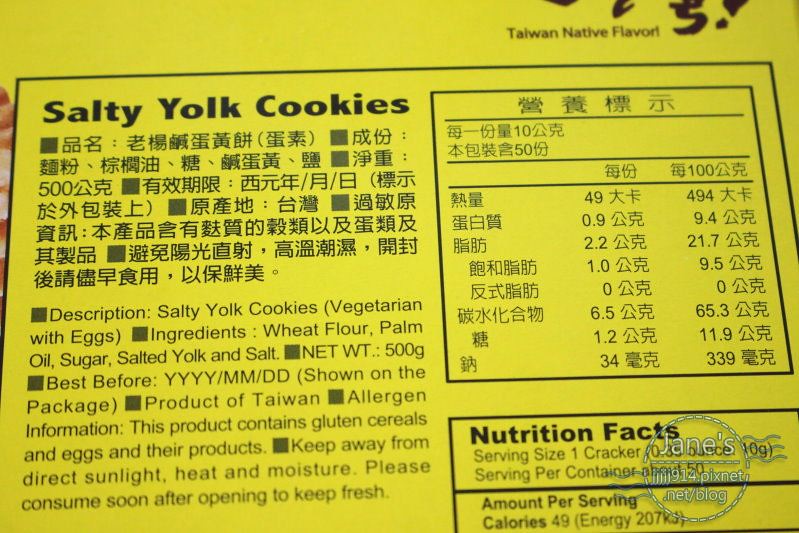This image showcases the back side of a yellow packaging box adorned with black text, prominently labeled "Salty Yolk Cookies" on the left side. At the top right corner, it states "Taiwan Native Flavor." Several Chinese characters, accompanied by English translations, describe the product. The package notes that these are "Salty Yolk Cookies" that are vegetarian, made with eggs. The ingredients listed include wheat flour, palm oil, sugar, salted yolk, and salt. The net weight is displayed as 500 grams, and a "Best Before" date is indicated as YYYY/MM/DD. 

This product is identified as being from Taiwan and carries allergen information, stating it contains gluten cereals and eggs and their derivatives. The packaging advises keeping the product away from direct sunlight, heat, and moisture, and to consume soon after opening to maintain freshness. 

To the right, there are two nutrition facts charts—one in Chinese and one in English. The English chart indicates that a serving size of one cracker is approximately 10 grams, with about 50 servings per container. Each serving provides 49 calories and 207 kilojoules of energy.